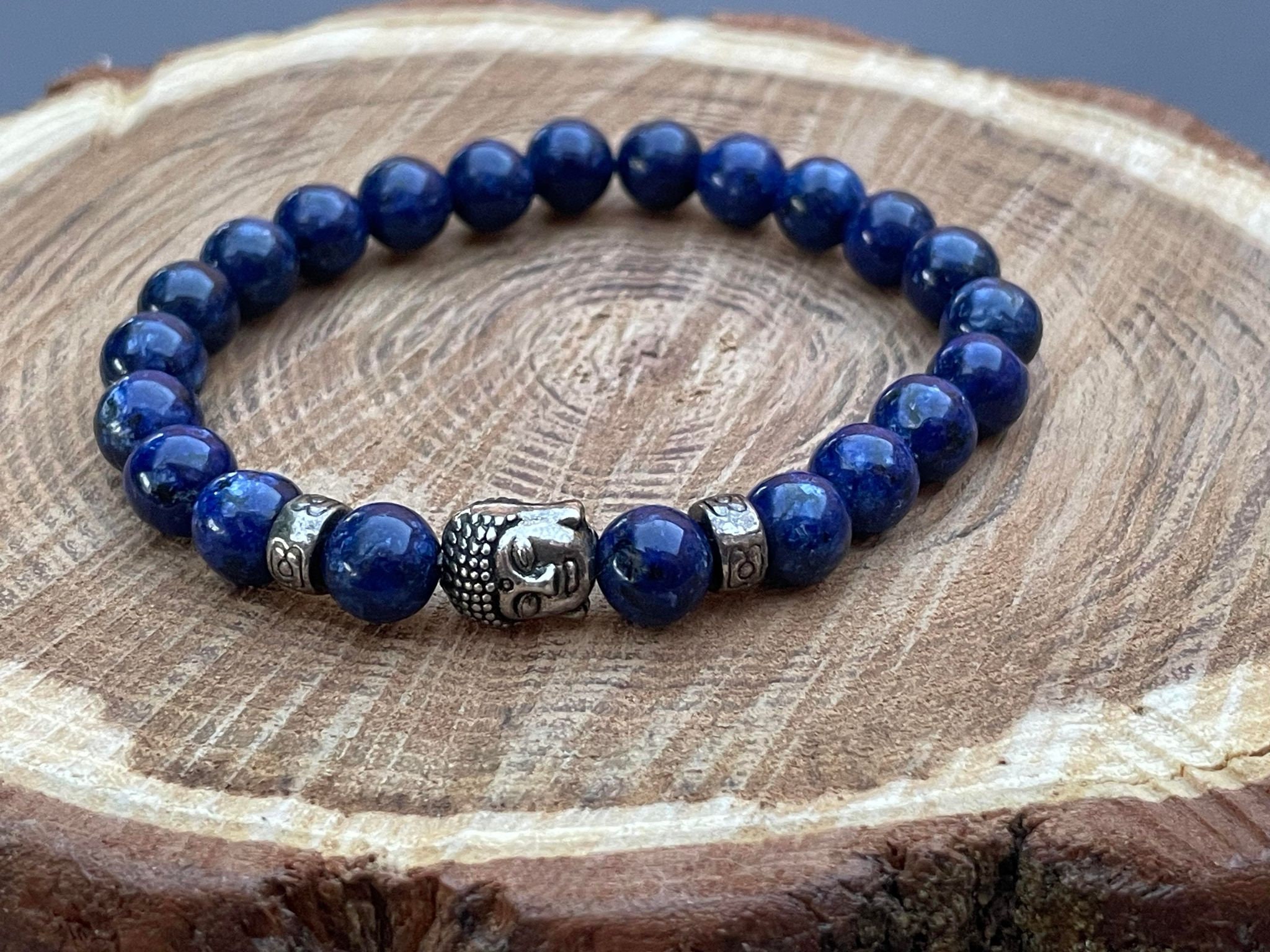This is a detailed color photograph of a bracelet placed on a round platform resembling a cross-section of a tree stump. The background is a solid blue color, bringing emphasis to the foreground. The platform showcases the natural rings of the wood, transitioning from darker brown bark on the outer edge to lighter brown and medium shades towards the center, highlighting the intricate details of the wood grain. The bracelet, predominantly composed of round, dark blue beads possibly made of lapis lazuli or sodalite, stands out strikingly against the wooden base. Interspersed among the blue beads are three silver-colored charms: two circular bands and one charm depicting a deity's face, adorned with round dots on its head, suggesting a Hindu influence. The combination of natural wood and the vibrant, shiny beads creates a visually compelling and richly textured image.